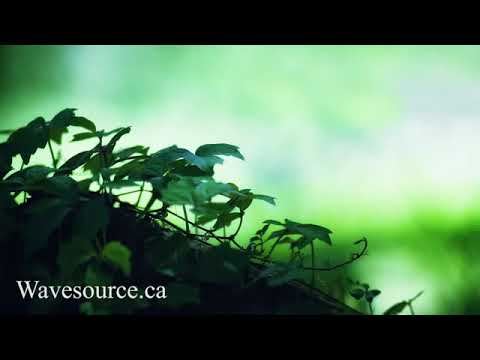This image appears to be a poster featuring a vibrant, outdoors green scene. The background is a diffused blend of mottled green and white, becoming darker towards the lower right edge. Two prominent black lines run horizontally across the top and bottom one-eighth of the poster. In the bottom left corner, the text "Wavesource.ca" is printed in white. The main focal point of the image is an ivy plant that extends diagonally from the upper left to the lower right. The dark green leaves and trailing vines add a dynamic and provocative element to the scene. The background is blurred with subtle hints of light blue and gray, suggesting an out-of-focus outdoor setting, possibly with sunlight filtering through. The plant appears to grow from or over a log situated diagonally in the lower portion of the image.